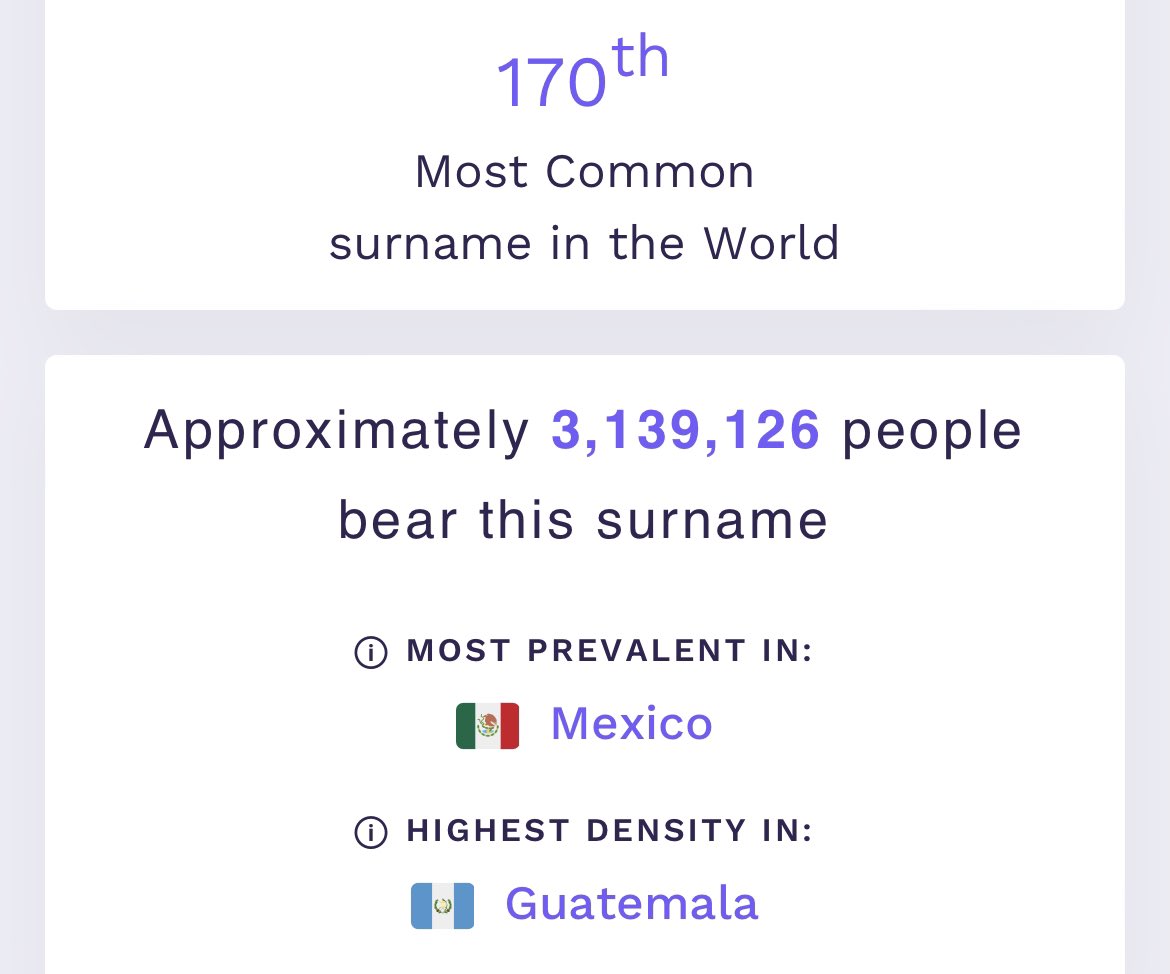This image is a cropped screenshot of a desktop highlighting statistical information about the prevalence and distribution of a specific surname globally. At the very top center of the image is the text "170TH" in light purple font, indicating the rank of this surname in terms of commonality worldwide. Directly below, in black text, are the words "most common surname in the world."

A blue horizontal bar separates this section from the subsequent information. Below the bar, the text continues in black but with a crucial number: "approximately 3,139,126," written in the same light purple font as before, indicating the number of people who bear this surname globally. Following this, the black text concludes with "people bear this surname."

Further down, there is information about the geographical distribution of this surname. It is noted that the surname is "most prevalent in" Mexico, where "Mexico" is displayed in the same light purple font, accompanied by a Mexican flag to its left. Lastly, the text indicates the "highest density in" Guatemala, with "Guatemala" also in the matching purple font, and the Guatemalan flag positioned to its left.